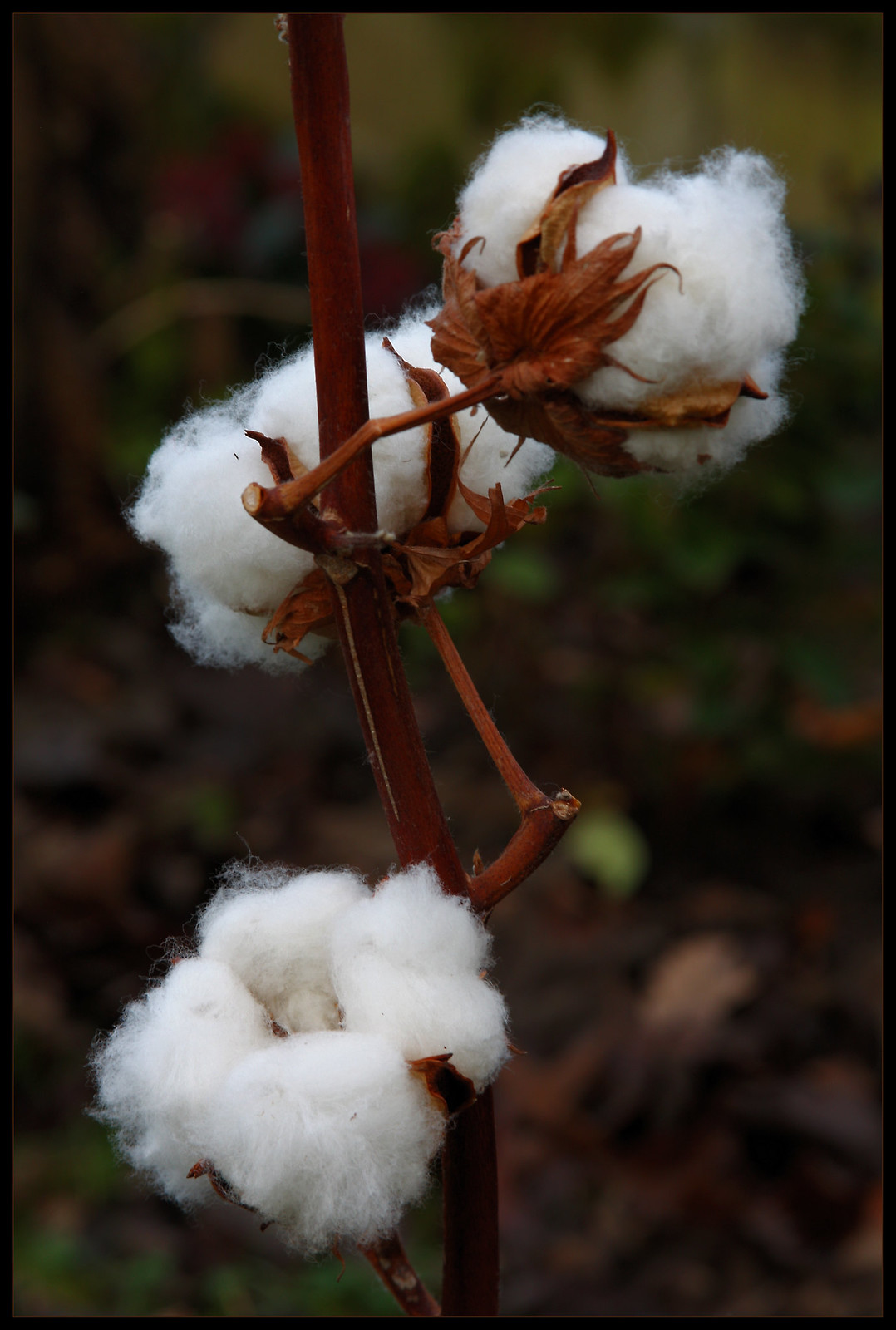The image is a vertically oriented, close-up photograph of a cotton plant, framed by a thin black border. The main stalk of the plant runs centrally from top to bottom, slightly offset to the left at the very top and curving towards the center as it approaches the bottom. The stem is a dark brown, almost dried-out in appearance, contrasting with the fresh and viable raw cotton buds.

There are three prominent tufts of budding cotton. Two are situated in the middle-top and middle-top-right, with one budding from a right-angled branch behind the main stalk, and another curving around to face away from the camera, thus revealing more of the leaves behind it. The third tuft is in the bottom-left section, emerging from a branch that appears from the bottom of the frame, showcasing its four distinct tufts.

The background is a blurred tapestry of brown and green, likely representing the surrounding natural environment. Its indistinct nature serves to emphasize the details of the cotton plant, making the stark whiteness of the cotton buds stand out prominently against the earthy colors.